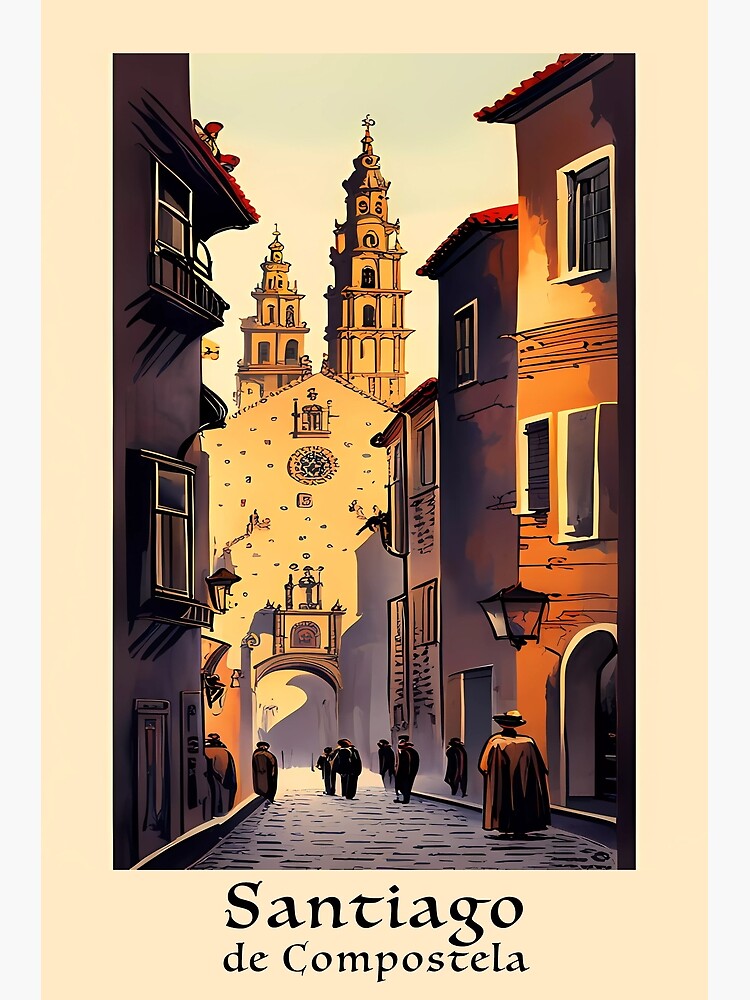This retro-designed illustration, possibly a modern rendition of a vintage aesthetic, depicts a historical street scene labeled "Santiago de Compostela" at the bottom in a beautiful font. The background is cream-colored, and the detailed image occupies the top four-fifths of the poster, showcasing a group of stylized figures wearing cloaks and hats. These figures, whose backs are turned to the viewer, walk in unison along a cobblestone path flanked by various colorful buildings. On the left, a two-story building with two windows appears in shadow, while on the right, a brightly lit, three-story building painted in rich tones of burnt orange, maroon, and yellow stands prominent. Further along the street, additional structures lead the eye towards a grand archway, which frames the towering spires of what appears to be a cathedral in the background. The muted color palette and intricate architectural details evoke a sense of historical Europe, potentially Spain, enhancing the scene's nostalgic and mysterious allure.